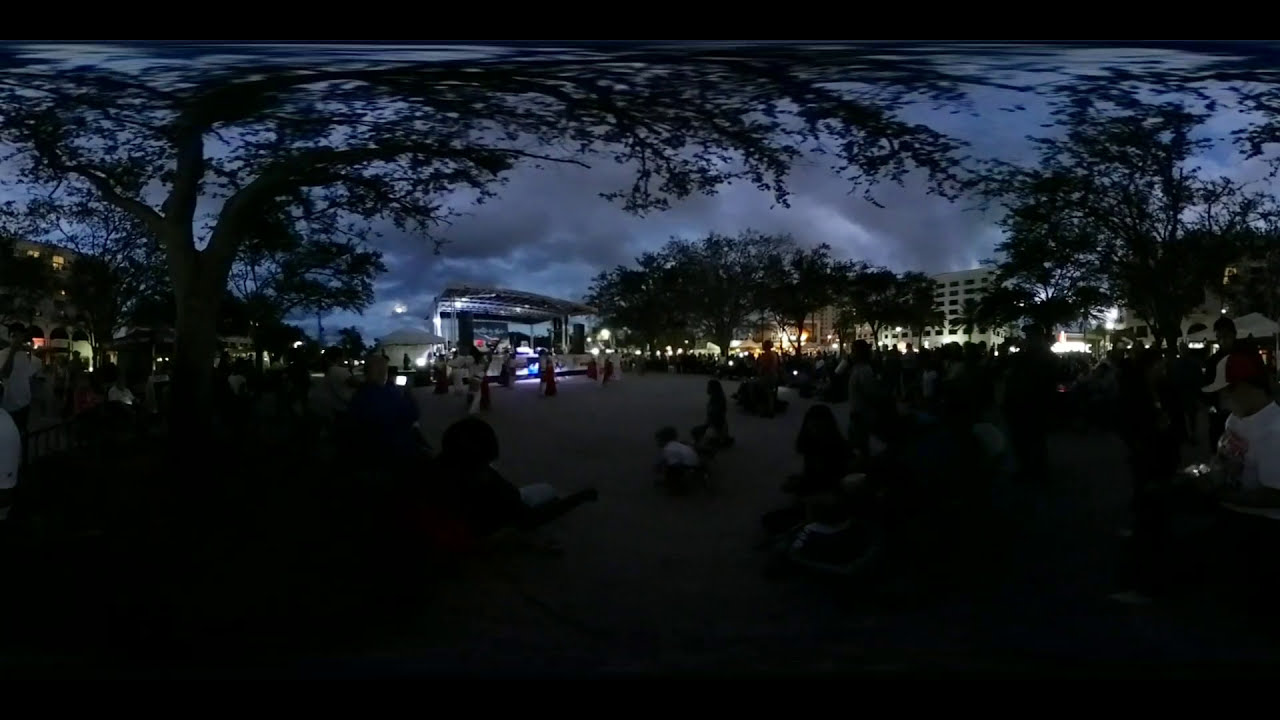This night scene captures an outdoor gathering in a park area. Central to the image is a small stage setup, with lights illuminating it despite the overall darkness. The stage, covered by an overhang, hosts some kind of performance, though the performers aren’t clearly visible. People are gathered around, most notably sitting on the left and right sides of the frame, with a few individuals discernible in the shadowed crowd. The ground near the stage seems to be grassy, and numerous trees are scattered throughout the park area. The sky is a dark blue, dotted with dark purple clouds, indicating it is night but not yet fully enveloped in darkness. In the distance, tall buildings loom behind the scene, adding to the urban landscape's ambiance. Lights in the background hint at a nearby parking lot or streets, adding a glow beyond the crowd. There is a notable tree on the left side of the image, its trunk branching out over the main open area where the performance takes place. The photo appears slightly warped at the top, possibly due to a 360-degree capture, emphasizing the trees that dominate the scene. Overall, this seems to be an outdoor concert or performance, possibly hosted in a large plaza or park setting, with the cityscape framing the background.